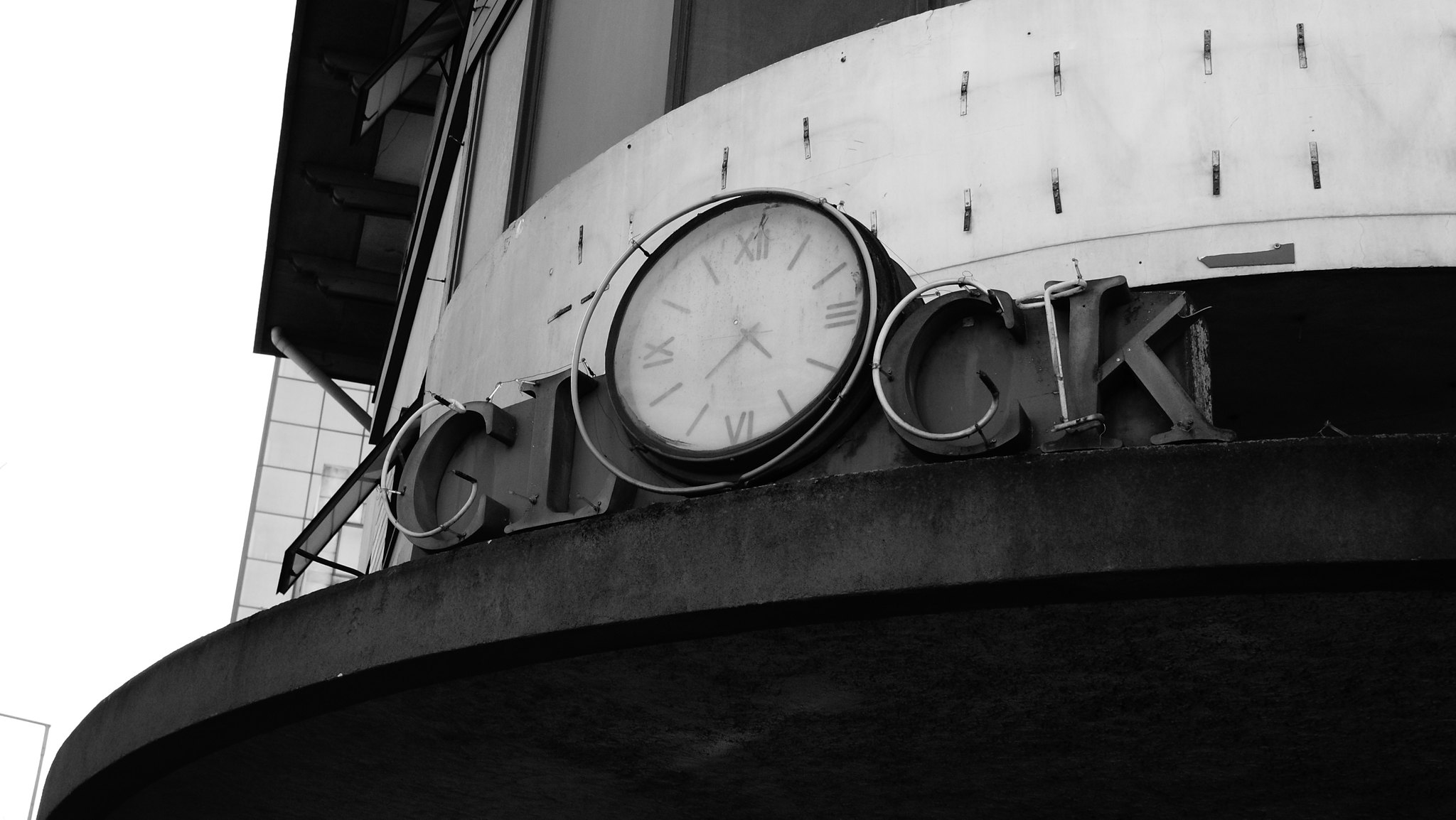In this horizontally oriented black-and-white photograph, we see an external view of a building facade. The focal point is a sign that spells out the word "CLOCK" in unlit neon letters, with the "O" uniquely designed as a prominent circular clock. This clock, twice the size of the other letters, features a white face with Roman numerals and indicates the time as 4:37. The surrounding architecture hints at an urban setting, with the lower left corner revealing another building adorned with glass windows. The interplay of the stark black-and-white tones adds a nostalgic, almost timeless feel to the image.